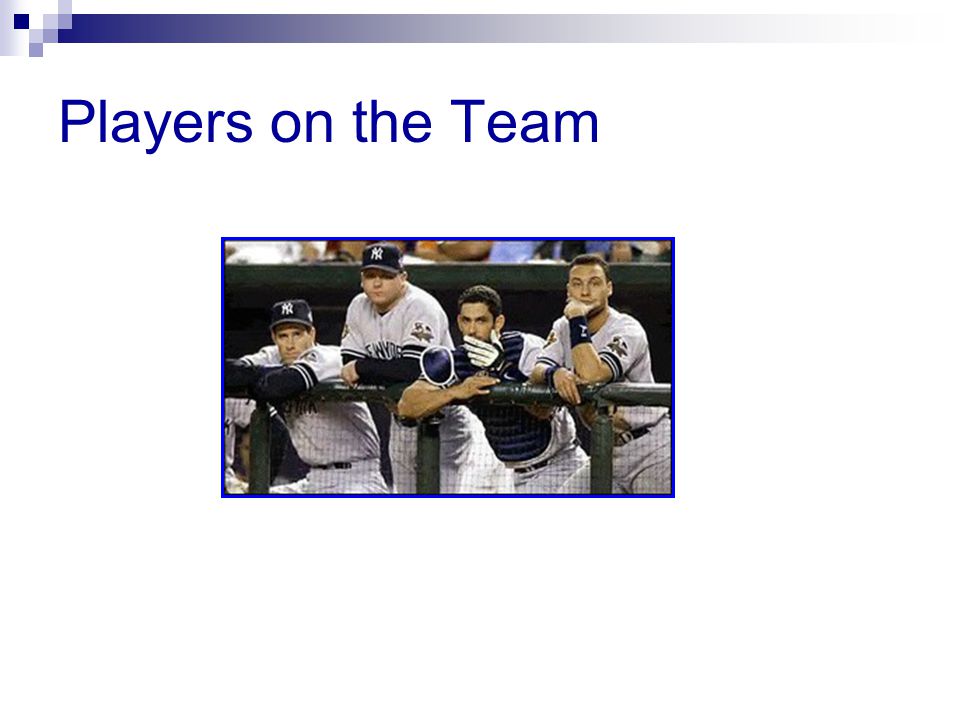The image, clearly presented in a PowerPoint-style format often used in educational settings, features a still moment from a New York Yankees baseball game. Positioned at the center of the screen, four white male players, including Derek Jeter, are showcased. They are dressed in the Yankees’ iconic white uniforms with blue accents, and two of them wear hats emblazoned with the team’s logo. The player on the right is identified as Derek Jeter. They are all leaning against a handrail or fence, looking upward as if watching the progression of the game, with a partially visible green wall and the indistinct forms of a crowd in the background. The image is bordered by a blue frame. Above the image, a gradient banner transitions from dark blue to light blue to gray and silver, adorned with a series of small colored squares on the left. Below the banner, blue text on a white background reads "players on the team," indicating the primary focus of the image.